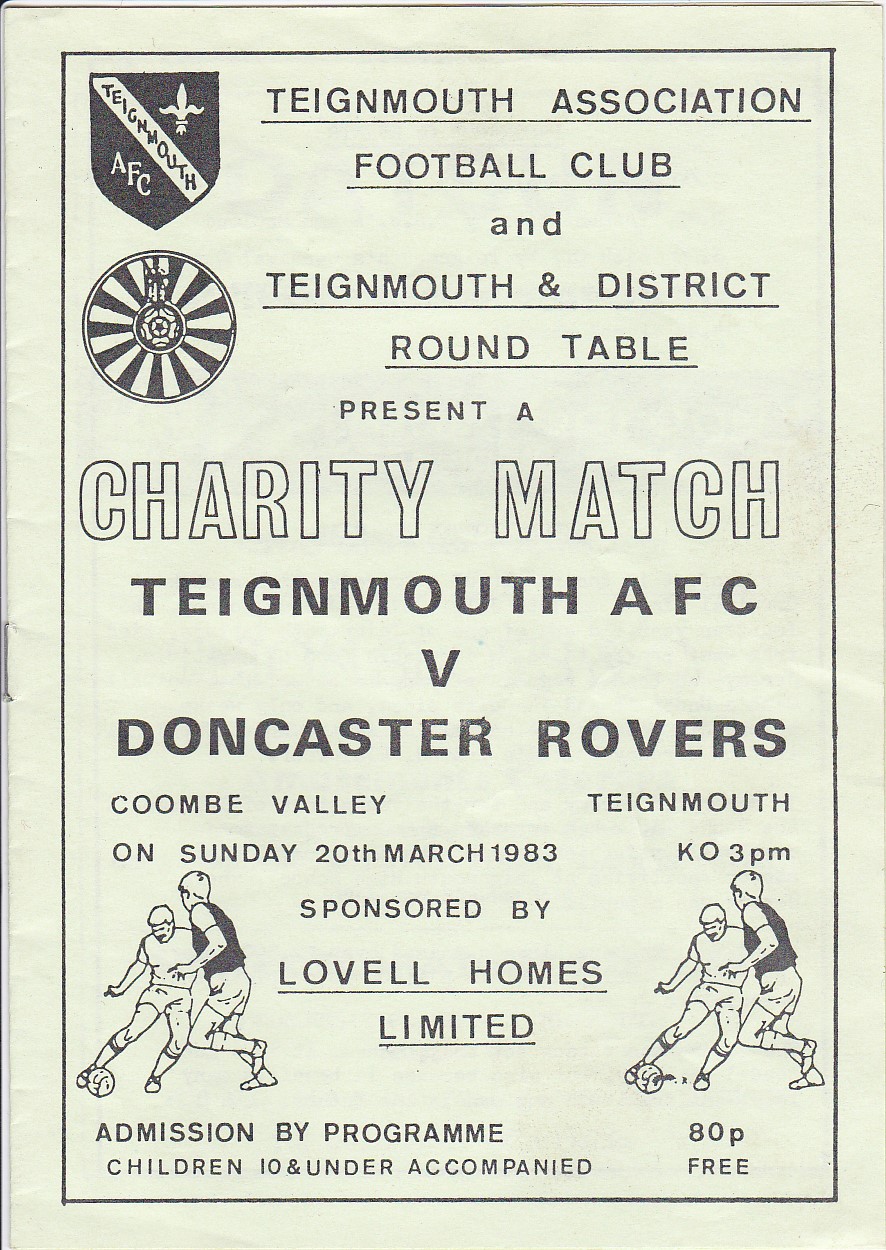This advertisement is for a charity soccer match organized by the Teignmouth Association Football Club in collaboration with the Teignmouth and District Round Table. It announces a match between Teignmouth AFC and Doncaster Rovers, to be held at Coombe Valley in Teignmouth on Sunday, March 20, 1983, with a kick-off at 3 PM. The event is sponsored by Lovell Homes Limited. The poster specifies that admission is by program, with children 10 and under allowed entry free when accompanied by an adult. The page features an emblem and a shield at the top, likely representing the club’s logo, and includes illustrations of soccer players in action on both sides of the lower part of the advertisement. The text is printed in a combination of black and gray against an off-white background.